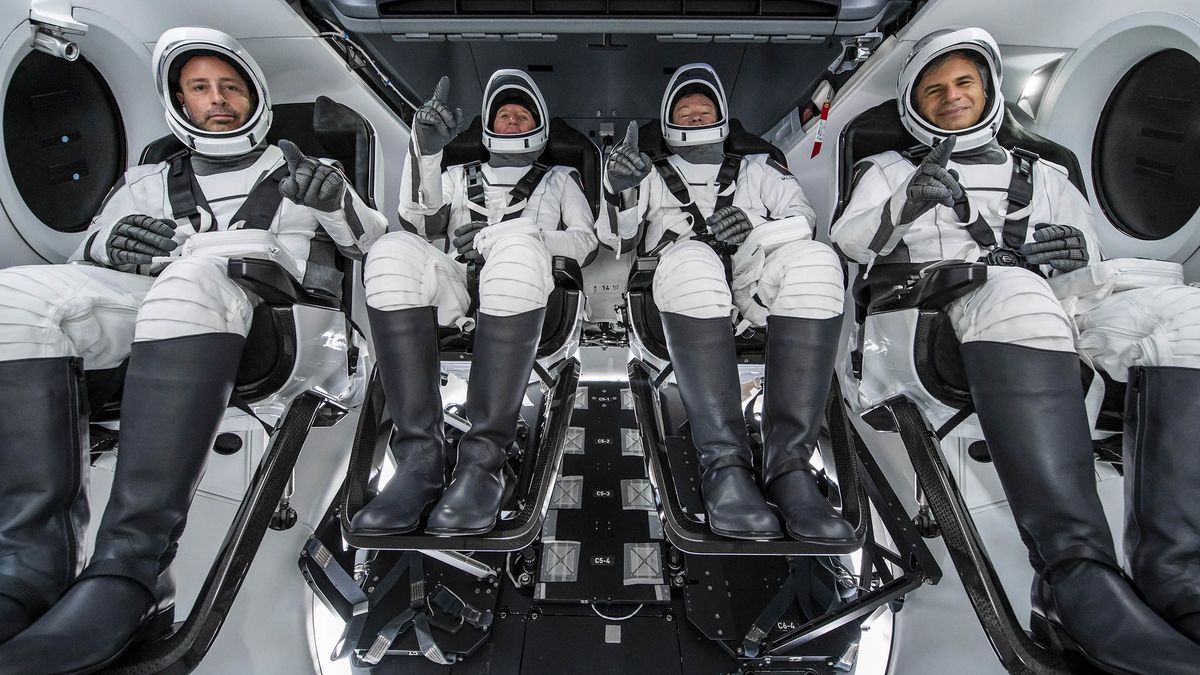This rectangular photograph depicts four astronauts seated side by side inside a spaceship. They are dressed in white and black space suits, complete with white helmets that have their visors raised, revealing their excited faces. Each astronaut is wearing knee-high black boots and white gloves. Their boots are propped up on small black footrests attached to their chairs. The astronauts are secured with safety belts and are all giving peace signs with one hand. The interior of the spaceship is predominantly white with circular black windows lining the sides, and the ceiling is also black.